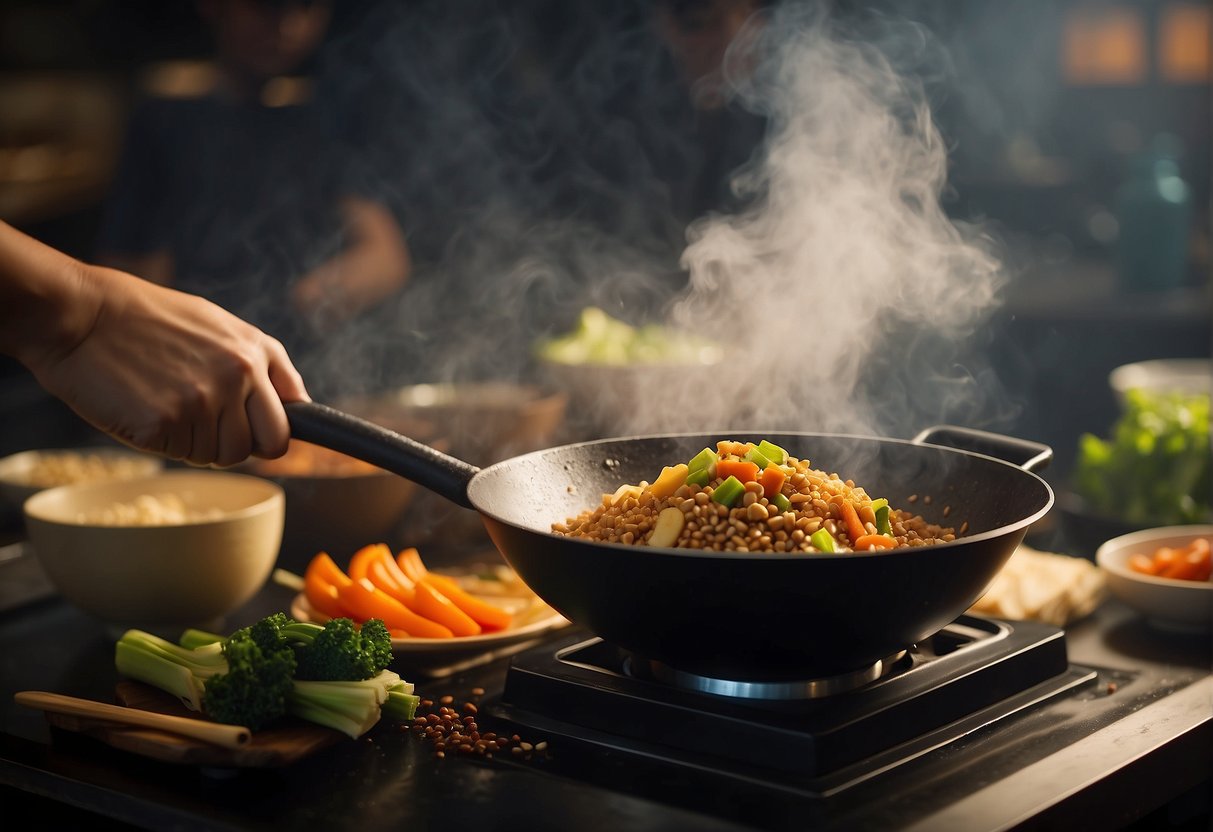The image showcases a culinary scene with a horizontally oriented photo of a person cooking a vibrant stir-fry. A hand, appearing from the left side of the frame and placed almost halfway down from the top, grips the black, round handle of a wok. The wok itself is positioned on a square black metal stove top, with steam rising from its colorful contents. Inside the wok, there is a mixture of various ingredients including soybeans, cubes of green and orange vegetables, and larger yellow beans. Surrounding the stove on a dark gray countertop are plates and bowls filled with different vegetables, such as carrots, chives, celery/broccoli, and lettuce, some of which are slightly blurred. The scene is detailed and dynamic, capturing the essence of a hot, fresh stir-fry being prepared. Notably, there is an AI-generated artifact of the hand holding the wok, which has six fingers, a common anomaly in artificial intelligence imagery.